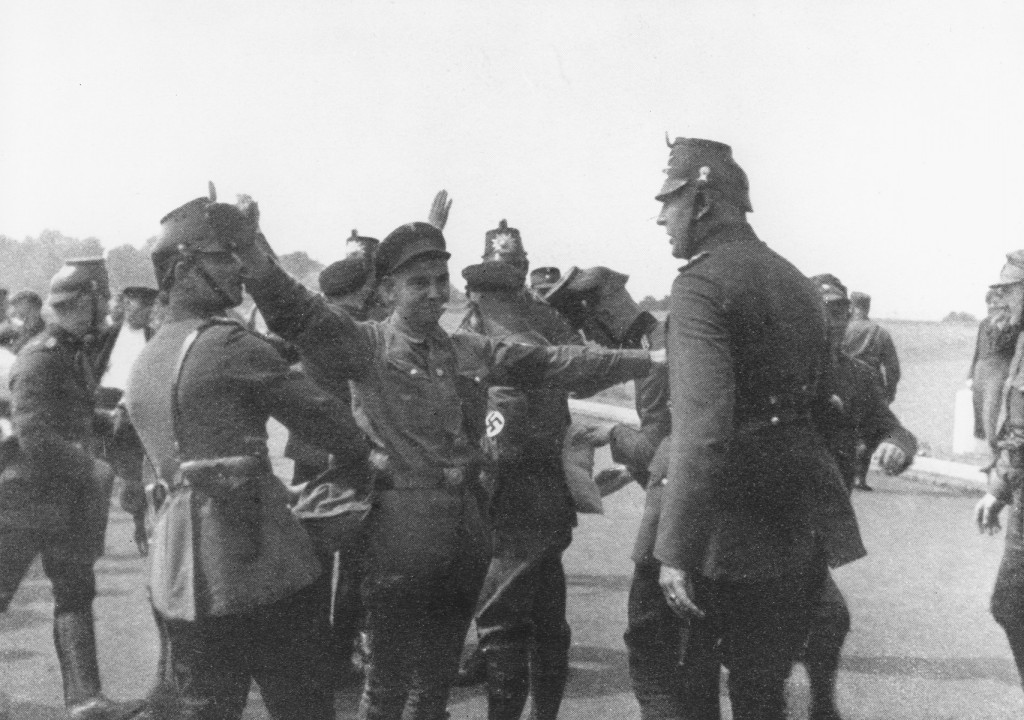This old black and white photograph depicts a group of Nazi soldiers clustered together in a countryside setting, likely during World War II. The men are dressed in military uniforms, with many wearing helmets or hats with neck straps. Distinctively, several soldiers have the swastika emblem visible on their sleeves. In the foreground, a younger soldier stands with arms outstretched, possibly indicating he's being searched or surrendering. This soldier's attire includes a hat and what might be a cigarette in his mouth. Beside him, an older, taller soldier, possibly in a position of authority, wears a ring on his finger and a similar neck strap helmet. Around 20-25 men populate the image, some seemingly engaged in conversation or movement, while others perform the "Heil Hitler" salute. The scene is set on a grey road with minimal background elements apart from a few distant trees and a white skyline. Despite a dense arrangement, the image subtly hints at interactions between soldiers, suggesting a scenario involving different or searching groups.